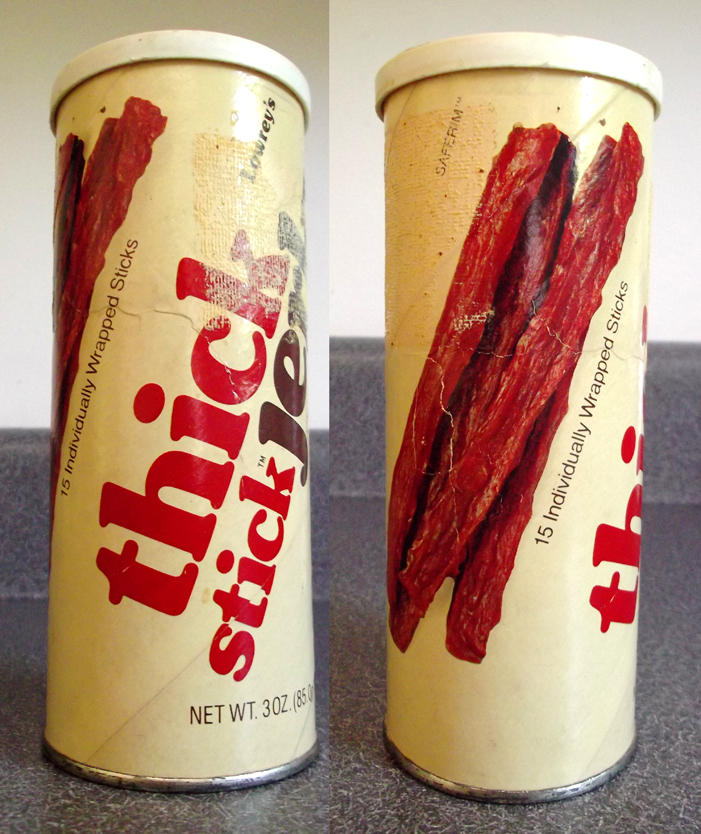This color photograph features two vintage-looking, beige paper canisters placed against a gray Formica countertop and a white wall, evoking a nostalgic feel. Each canister is topped with a white lid and adorned with vibrant color images of meat sticks. The prominent text on the canisters is in red and brown, advertising "Thick Stick Jerky" by Lowrey's. Each canister contains 15 individually wrapped sticks with a total net weight of 3 ounces. The overall design and typography reflect an older era, making the canisters appear classic and timeless.